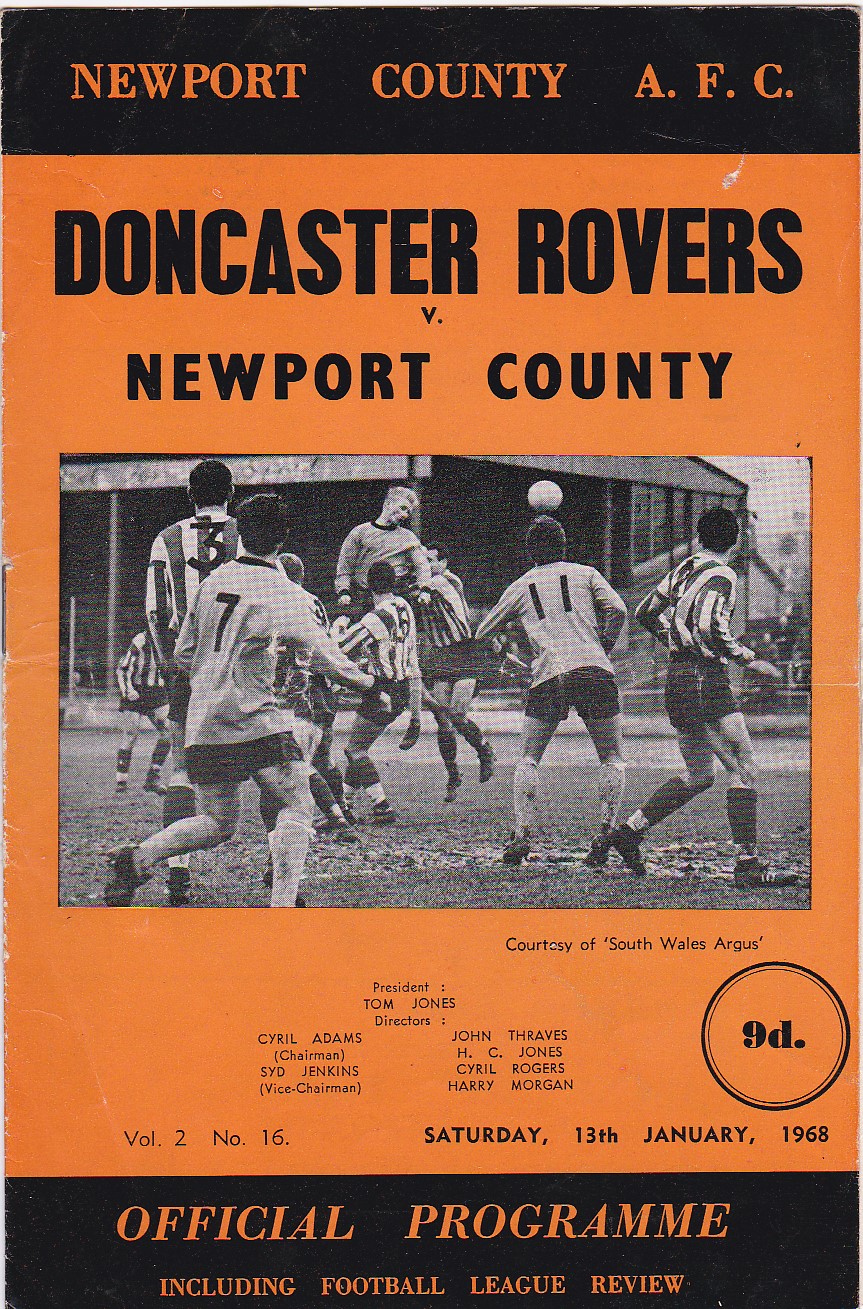This image is a color photograph of a program cover meant to be distributed to spectators at a soccer match. The background of the cover is primarily orange, with key sections defined by black rectangles. At the top is a black bar with orange text that reads "Newport County AFC." Just below this, in bold black text against the orange background, it reads "Doncaster Rovers v. Newport County." The central feature of the cover is a black and white photograph showing around 10 soccer players in action on a muddy field, with a visible soccer ball. The players are wearing differently styled jerseys, some in solid white and others in white with stripes. Beneath the photograph, additional text reads "Courtesy of South Wales Argus." Further below are the names of notable individuals, including President Tom Jones, Director Cyril Adams, Chairman Sid Jenkins, Vice Chairman John Thraves, HT Jones, Cyril Rogers, and Harry Morgan, as well as details like "Volume 2, Number 16, Saturday 13th, January 1968, 9-D." At the very bottom, another black rectangle contains orange text that states "Official Program, including Football League Review."